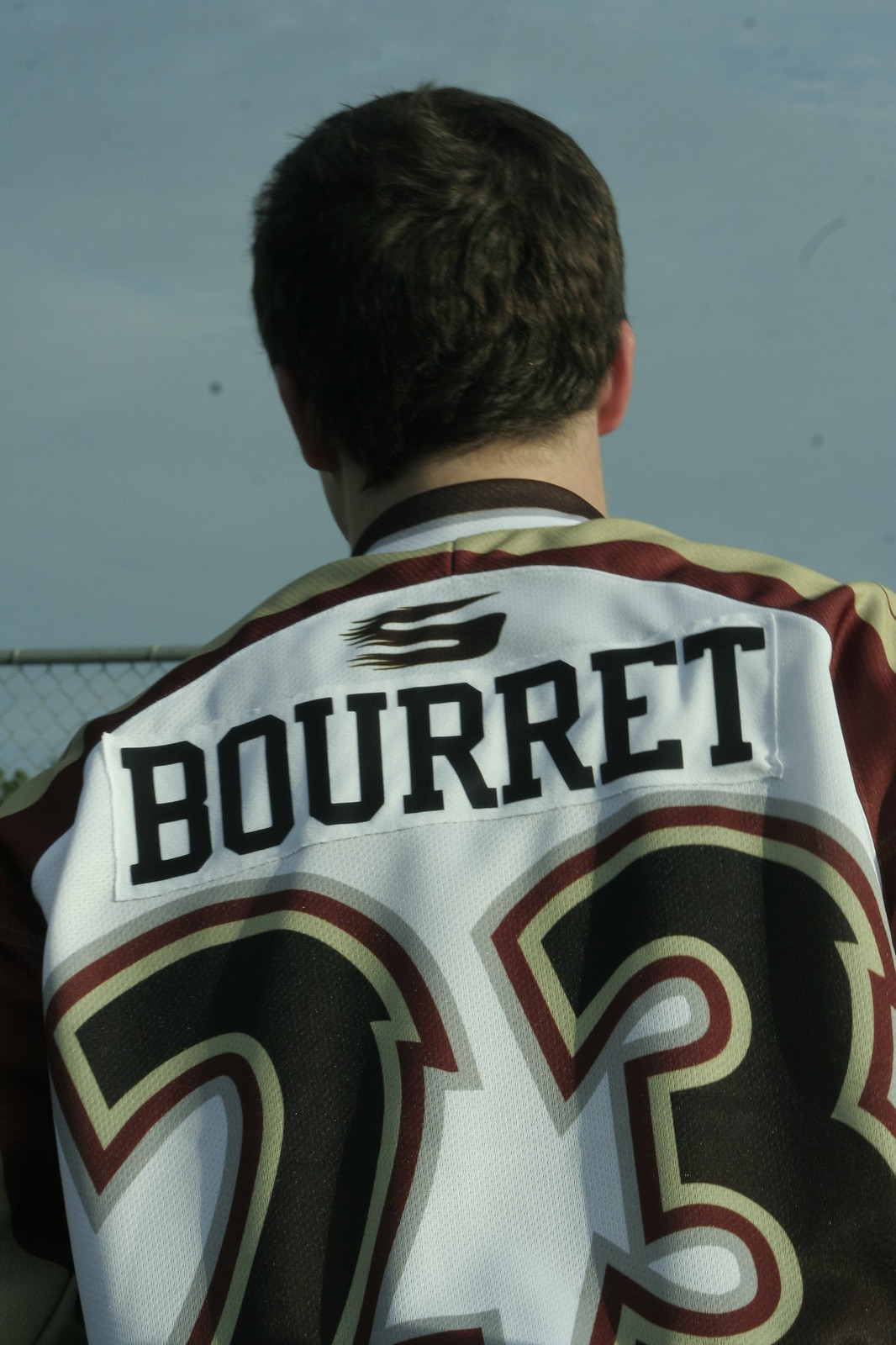The image portrays a young man standing with his back to the camera, wearing a sports jersey adorned with the name "Barrett" and the number "23." His short-cropped black hair is visible, and he does not wear a helmet, suggesting an off-field moment. The jersey features the colors burgundy, gold, white, black, and tan, with intricate, almost fire-like embellishments on the number "23." The setting appears to be outdoors, characterized by an overcast sky and a chain-link fence partially visible in the upper corner. The dreary lighting and overall composition imply a daytime scene, yet slightly dark or overcast. The ambiguity of the jersey's specific sport—whether hockey, soccer, or football—remains, but the details provided paint a vivid picture of the individual and his attire.